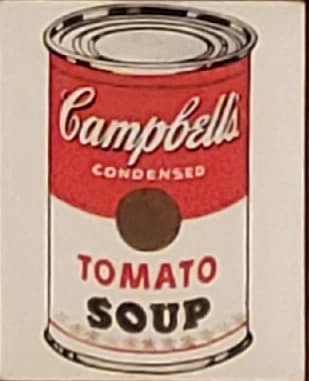The image is a vertically-oriented, rectangular painting of a Campbell's Condensed Tomato Soup can, reminiscent of Andy Warhol's iconic series. The can has a metallic lid at the top and a label that wraps around its body. The upper section of the label is red with the cursive word "Campbell's" in white, followed by the small word "Condensed" beneath it. A round, brown medallion intersects the red and the lower white section of the label, creating a visual focal point. In the white section, "Tomato" is written in red and "Soup" in bold black lettering. A thin red line encircles the can near the bottom, just above a small metallic rim. The artwork captures the essence of a vintage advertisement and is set against a plain beige background, emphasizing its nostalgic and classic design.